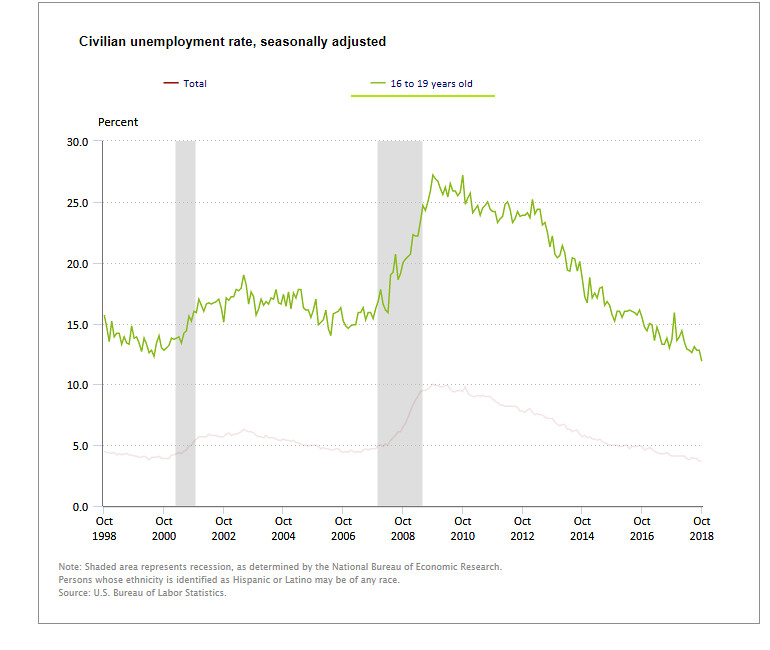This is a detailed graph titled "Civilian Unemployment Rate Seasonally Adjusted." The graph covers the period from October 1998 to October 2018, marked at two-year intervals along the horizontal axis. The vertical axis, labeled "Percent," ranges from 0% to 30% in increments of 5%. 

Two trend lines are depicted: a red line representing the total civilian unemployment rate and a green line representing the unemployment rate for individuals aged 16 to 19 years. The green line is more jagged and consistently higher than the red line. It starts around 15%, peaks at approximately 28% in October 2009, and then declines back to around 15%. Meanwhile, the red line starts at 5%, rises to about 10% around the same peak period, and then also declines.

The background includes shaded areas indicating recession periods as determined by the National Bureau of Economic Research. Additional notes mention that persons identifying as Hispanic or Latino may belong to any race, with data sourced from the U.S. Bureau of Labor Statistics. The graph is set against a plain white background, making the colored trend lines and shaded recession periods stand out clearly.